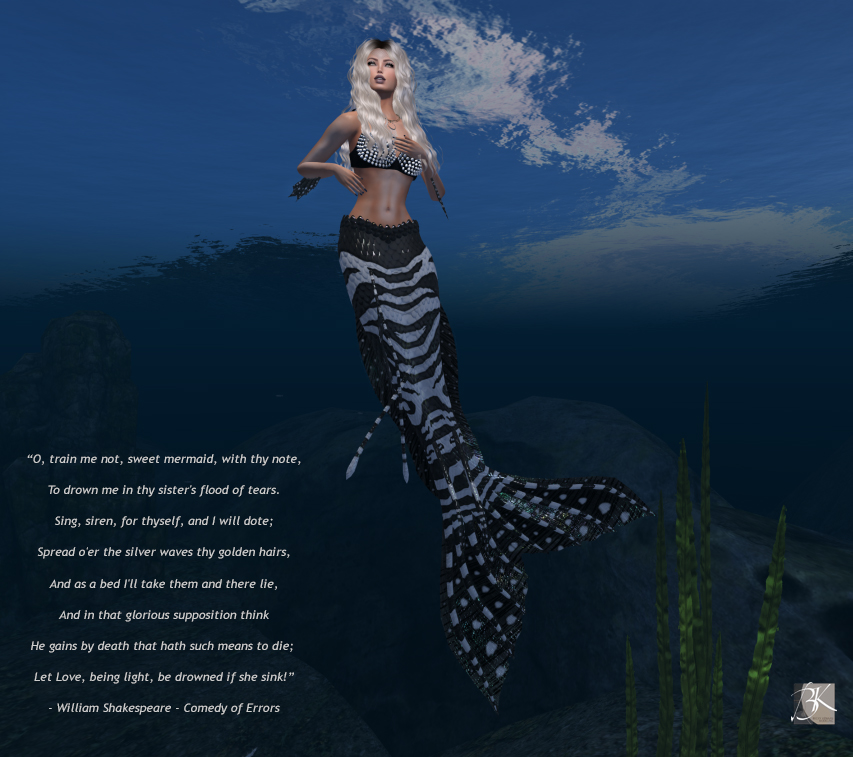The image resembles an album cover and depicts a detailed 3D render of a cartoon-style mermaid underwater, reminiscent of graphics seen in platforms like Second Life. The mermaid has a striking appearance with long, wavy blonde or silvery hair, featuring darker roots. She wears a bikini that appears studded or embroidered with silver jewels, adding to the shimmering effect. The mermaid's tail is intricately designed with a black and white or blue and black patterned appearance, reminiscent of a lobsters’ tail with delicate fin points or resembling the tails of angelfish or zebrafish. The underwater scene reflects the sky above the water's surface, enhancing the fantasy element of the image. In the bottom right corner, there is a white text overlay of a Shakespearean quote from "Comedy of Errors," which reads: "Oh, train me not, sweet mermaid, with thy note to drown in thy sister's flood of tears. Sing siren for thyself, and I will dote. Spread o'er the silver waves thy golden hairs, and as a bed I'll take them there and lie, and in that glorious position think he gains by death that hath such means to die. Let love, being light, be drowned if I sink." Additionally, there is a logo reading "BK" in the same corner. The background transitions between shades of blue and dark blue, adding depth and mystery to the underwater setting.